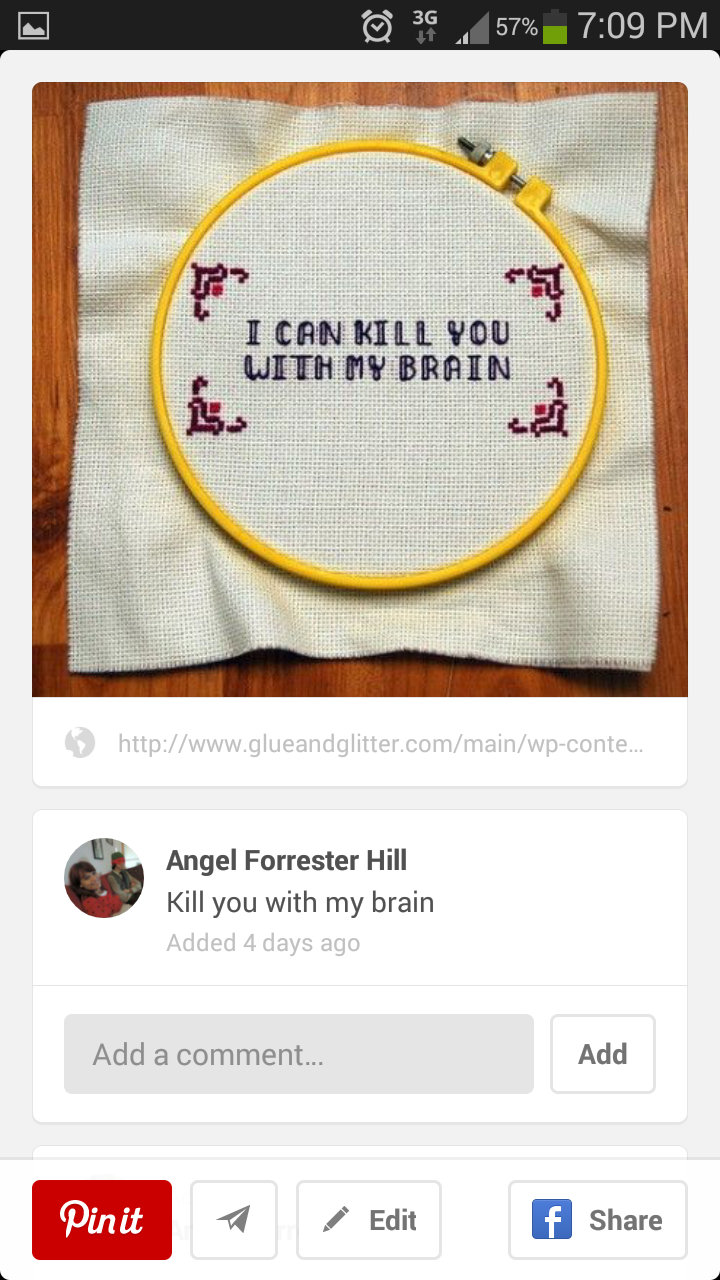The image displays a screenshot on a mobile phone featuring a white knitted square with blue yarn text that reads "I can kill you with my brain." The knitted piece is held taut by a yellow circular ring with a screw. The screenshot, likely from Pinterest, shows details in the upper-left corner, including an image logo and the website "gloonglitter.com." The screen also details "Angel Forest Hill" at the bottom, indicating the item's title with a note stating it was added four days ago. Additional screen elements include a battery symbol at 57%, a 3G connection, and a timestamp of 7:09 PM. The user interface shows options such as "Add comment," "Pin it," "Edit," and a Facebook share button. A truncated website URL, "www.glueandglitter.com/main/WPcon...", is also visible.